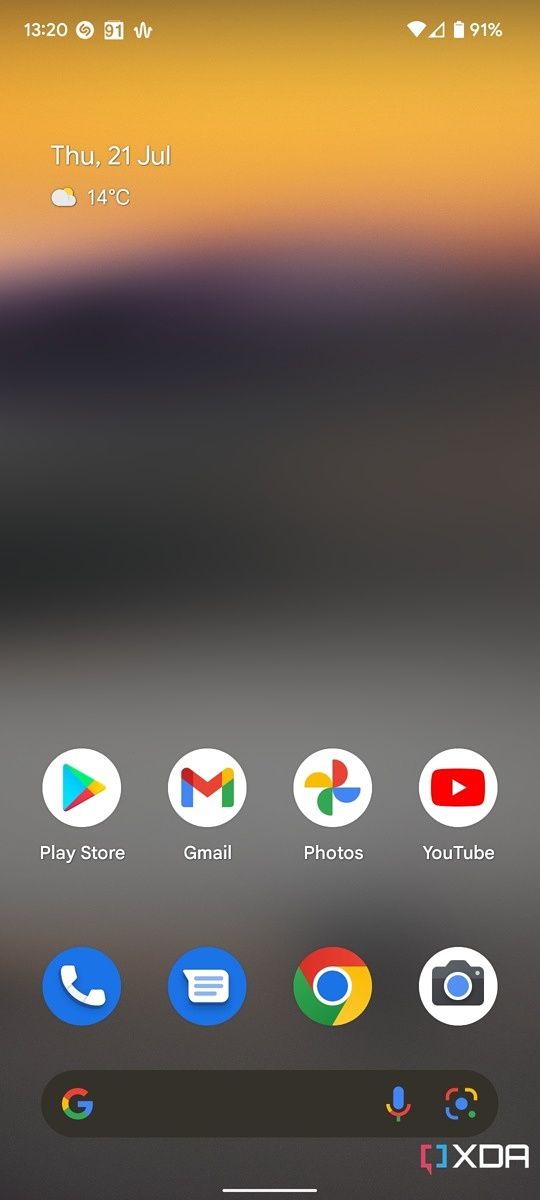A detailed shot of a phone's home screen showcasing a colorful, blurred gradient wallpaper transitioning from orange at the top to various shades of purple and gray, culminating in a medium gray at the bottom. The time displayed is 13:20, with a small icon on the left resembling a stylized "S" made out of a "C" and a backward "C," possibly a Spotify logo. The screen also features a battery indicator on both the left and right, each showing 91% with the left side also displaying a heart monitor-like squiggle. Wi-Fi strength is low, indicated by one out of four bars. The date reads Thursday, the 21st of July, and the temperature is 14 degrees Celsius. App icons for the Play Store, Gmail, Photos, and YouTube are aligned near the bottom. Above them are icons for Phone, Texting, Chrome, and Camera, accompanied by the Google search bar with a "G," microphone, and image search icon. At the bottom-right corner, the QXDA icon features a thought bubble split into red and blue halves.